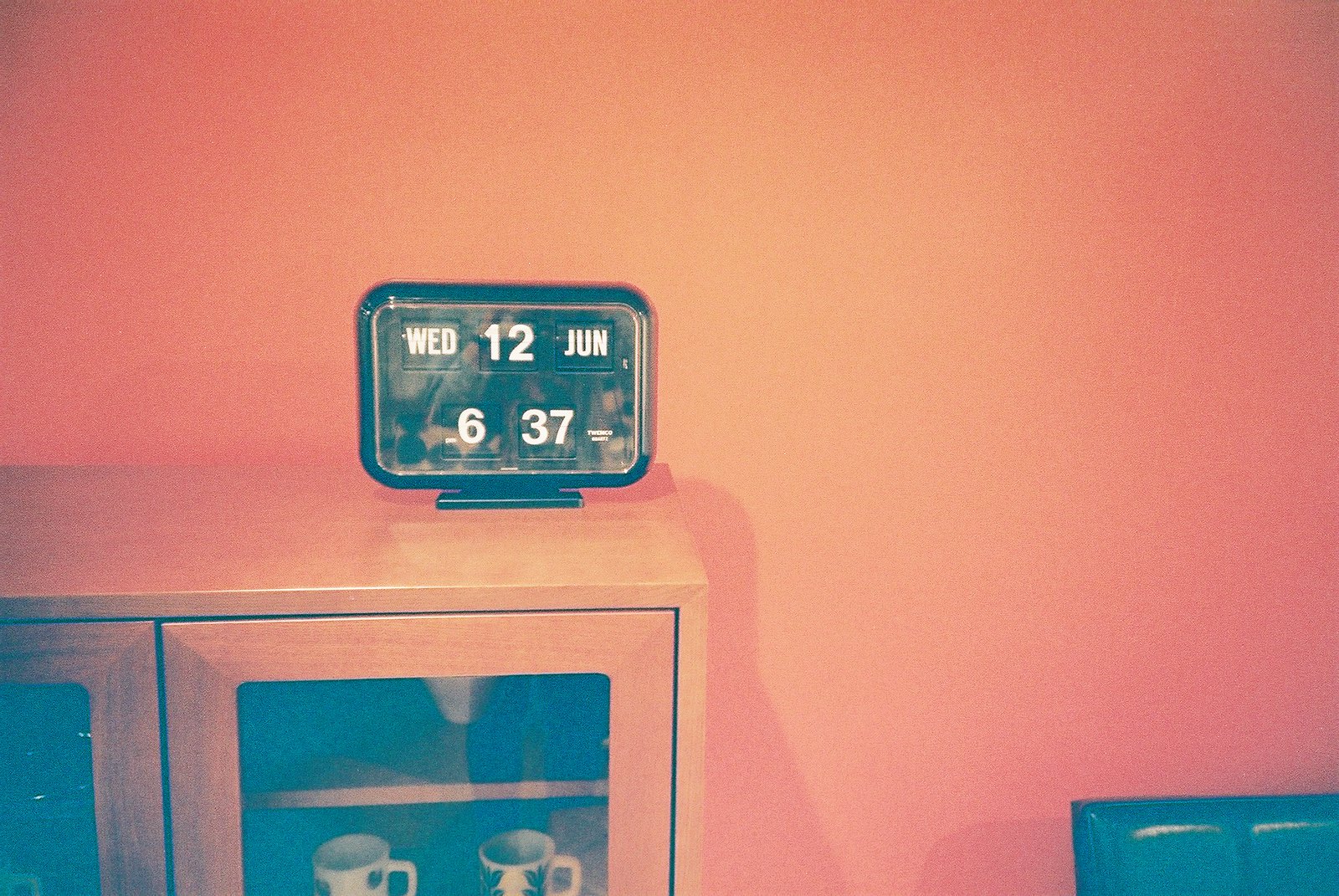In this photograph, a sleek, black rectangular clock with rounded edges sits atop a brown cabinet with glass doors. The polished clock, displaying the date "Wednesday, 12 June" and the time "6:37" in clear, white text, stands out against the warm, orange-painted wall in the background. Beneath the clock, through the cabinet's glass doors, you can spot two distinct white coffee mugs, each adorned with unique designs. Adding a subtle touch of contrast, the bottom left corner of the image reveals a fragment of another piece of furniture, hued in a soft blue tone.